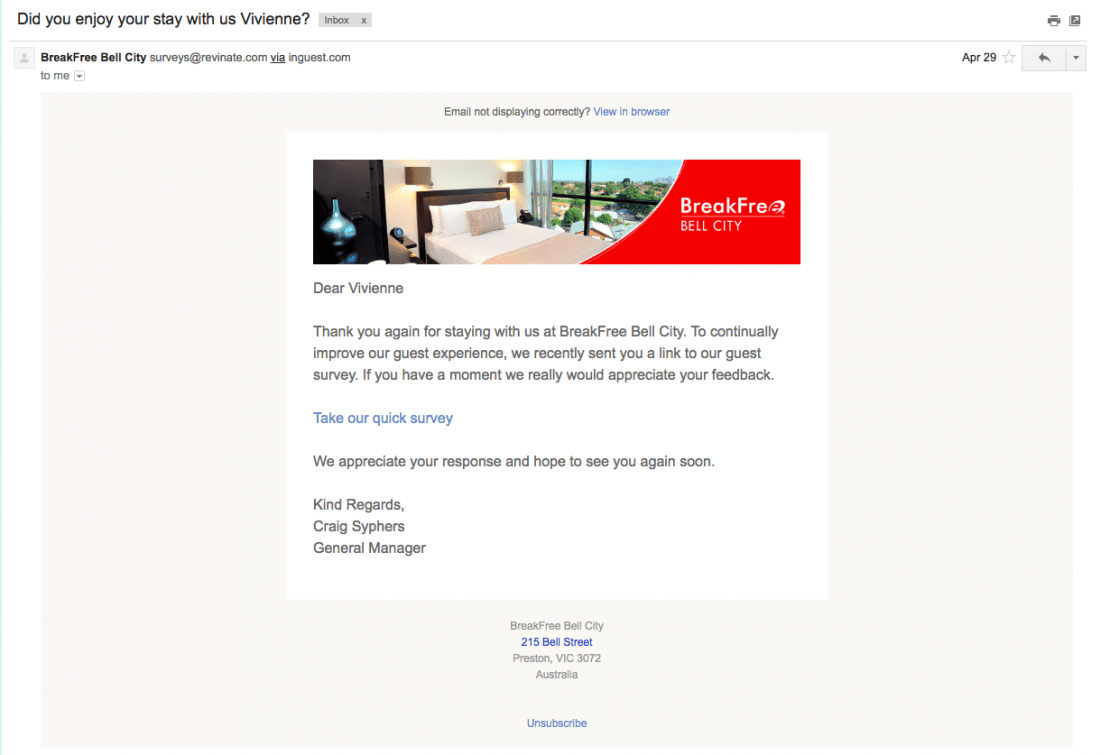Screenshot Description: 

The screenshot captures an email layout with clear delineation of various elements set against a predominantly white background. At the top left, black text reads, "Did you enjoy your stay with us at Vivienne?" Accompanying this text to the right is a medium gray square containing dark gray text that says "Inbox," followed by a dark gray "X" icon.

To the far right of the header, there are two more icons: a dark gray printer icon and a dark gray square with a white arrow pointing upwards and to the right at a 45-degree angle. Below this header, a thin light gray line serves as a separator.

In the section beneath this line, the layout begins with a light gray square on the far left, holding a medium gray generic profile picture icon. To the right of this square, bold black text reads, "Break Free, Bell City." Adjacent to this text, medium gray text displays, "Surveys at Revenate.com," followed by the underlined and gray "Via InGuest.com." At the far right, the date "April 29" is displayed in black, flanked by a light gray star icon. Continuing to the right, there's a light gray box with a medium gray arrow pointing to the left, attached to another narrower box with a dark gray arrow pointing downwards.

Below these elements, under the bolded text, gray text states, "To Me," and to its right, a white box outlined in light gray with a light gray arrow pointing down.

The body of the email has an eggshell white background. Centrally positioned is a white square featuring a photograph of a hotel bedroom. Connected to the photo on the right by a curving white line is a red section, extending to the same pane as the photograph, with white text that reads, "Break Free." Beneath this, in thinner text, "Bell City" is displayed. 

Underneath this visual section, gray text on the white background conveys the email's message: "Dear Vivienne, thank you for staying with us at Break Free, Bell City. To continually improve our guest experience, we recently sent you a link to our guest survey. If you have a moment, we really would appreciate your feedback."